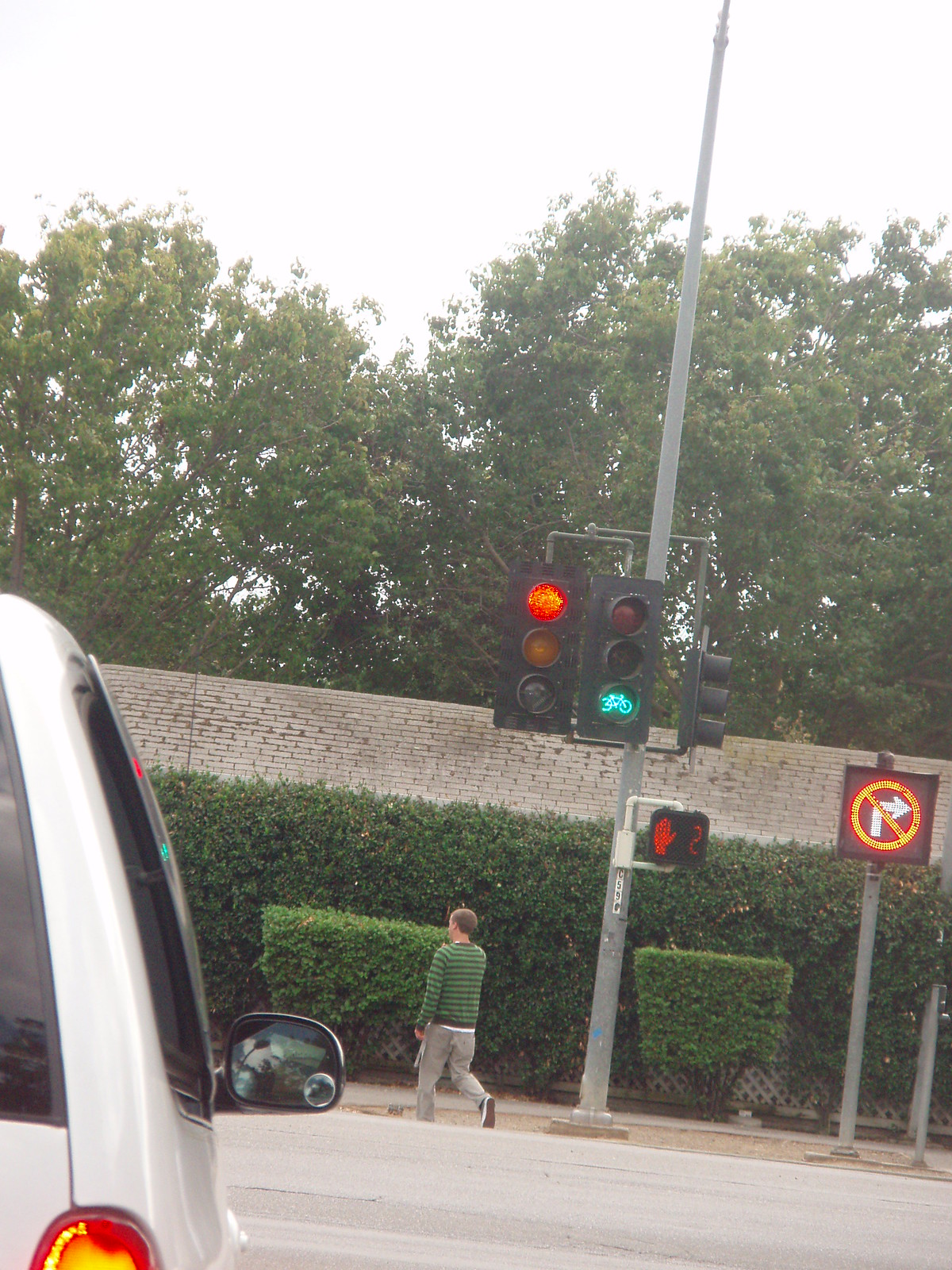The image depicts a bustling crosswalk at a busy intersection during the daytime. Dominating the scene are several traffic signs and signals, including a "no right turn" sign with a white arrow inside an orange circle with a line through it, mounted on a large silver post to the left. There are three streetlights with different signals: one displays a red light, another a green light specifically for bicycles, and the third light's status is obscured as it faces away. Additionally, a "don't walk" sign with an illuminated orange hand and a countdown showing the number two is visible lower down the post. Prominently featured in the foreground is part of a white vehicle, including the rear-view mirror and what could be the taillight on the left edge of the frame. Across the intersection, a person clad in a green and black horizontally striped shirt, khaki pants, and tennis shoes is seen crossing the street, approaching the sidewalk. Complementing the urban landscape are bushes lining the far side of the street, contributing to the scene's depth and detail.